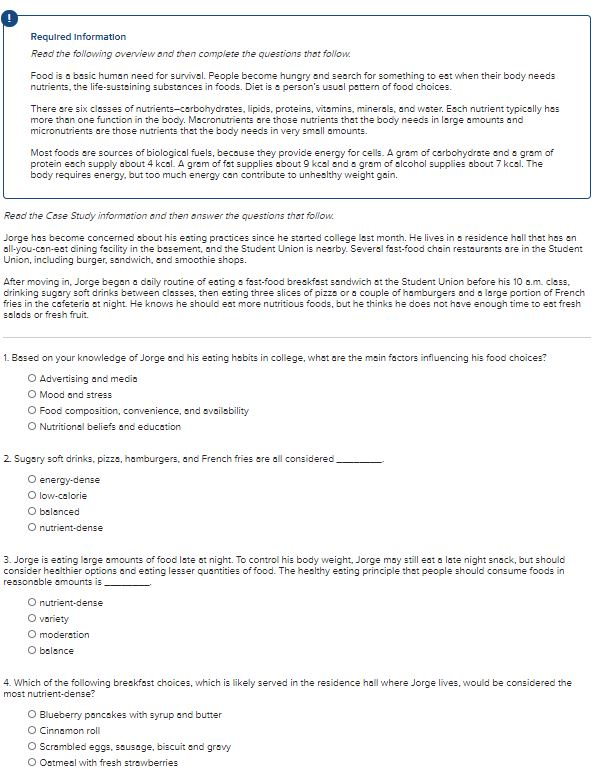The image features a shaded blue rectangle that encompasses a paragraph of text, marked by a standard warning symbol in the top-left corner. The heading at the top reads "Required Information" in blue. The initial lines of the text instruct the reader to "read the following overview and then complete the questions that follow." The content provides general information about the role of food in providing energy to the human body, noting that while a certain amount of energy is necessary, excessive consumption can lead to weight gain.

Following this introductory paragraph, the text prompts readers to "read the case study information and then answer the questions that follow." Below this, a paragraph details the case study, which is succeeded by a fine gray line. A set of multiple-choice questions appears thereafter. 

1. **Question One**: Based on your knowledge of George and his eating habits in college, what are the main factors influencing his food choices? Four possible options are provided for selection.
2. **Question Two**: Sugary soft drinks, pizza, hamburgers, and French fries are all considered... with four potential answers to choose from.
3. **Question Three**: George is eating large amounts of food late at night to control his body weight. The statement suggests that George may still eat a late-night snack but should consider healthier options and smaller portions. The healthy eating principle emphasized here—consuming foods in reasonable amounts—has four possible answers to select from.
4. **Question Four**: Among the breakfast choices available in George's residential hall, which one would be considered the most nutrient-dense? Again, there are four options listed for selection.

Each question is designed to assess the reader's comprehension and application of healthy eating principles as outlined in the case study and overview text.